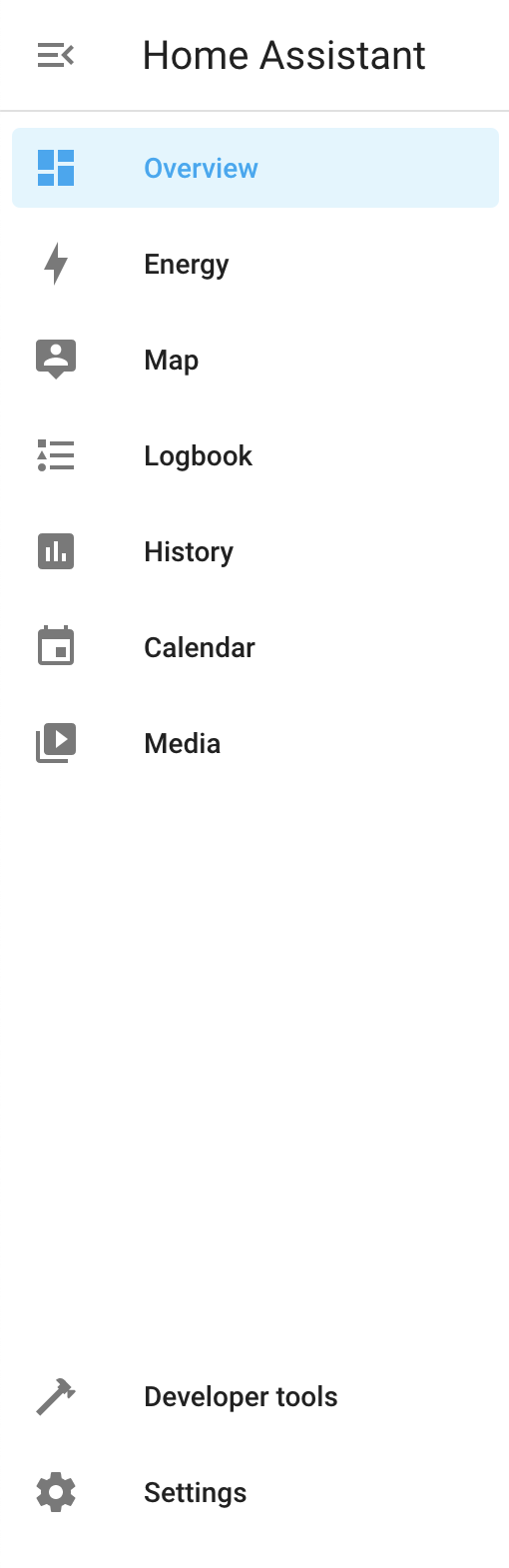The image displays a detailed settings page from the Home Assistant platform, featuring a user-friendly interface. At the top, the header is labeled "Home Assistant," accompanied by navigation arrows pointing right. Below this, several tab options are available for navigation:

1. **Overview** - Highlighted in blue, indicating it is the currently active tab. This section contains multiple windows for a comprehensive view.
2. **Energy** - Represented by an icon of a lightning bolt.
3. **Map** - Indicated by a pinpoint icon with a human outline.
4. **Logbook** - Shows a variety of lines and geometric shapes, including squares, triangles, and circles.
5. **History** - Illustrated with a gray bar graph icon.
6. **Calendar** - Marked by a calendar icon outline.
7. **Media** - Represented by a gray square with a play button inside.

Below these options are advanced sections:

8. **Developer Tools** - Denoted by an outline of a hammer in gray.
9. **Settings** - Represented by a gray gear wheel icon.

The overall background of the settings page is predominantly white, featuring gray-colored text and various icons. The layout and design are typical for a settings interface found within an app or on a web page, ensuring ease of navigation and a clean visual experience.